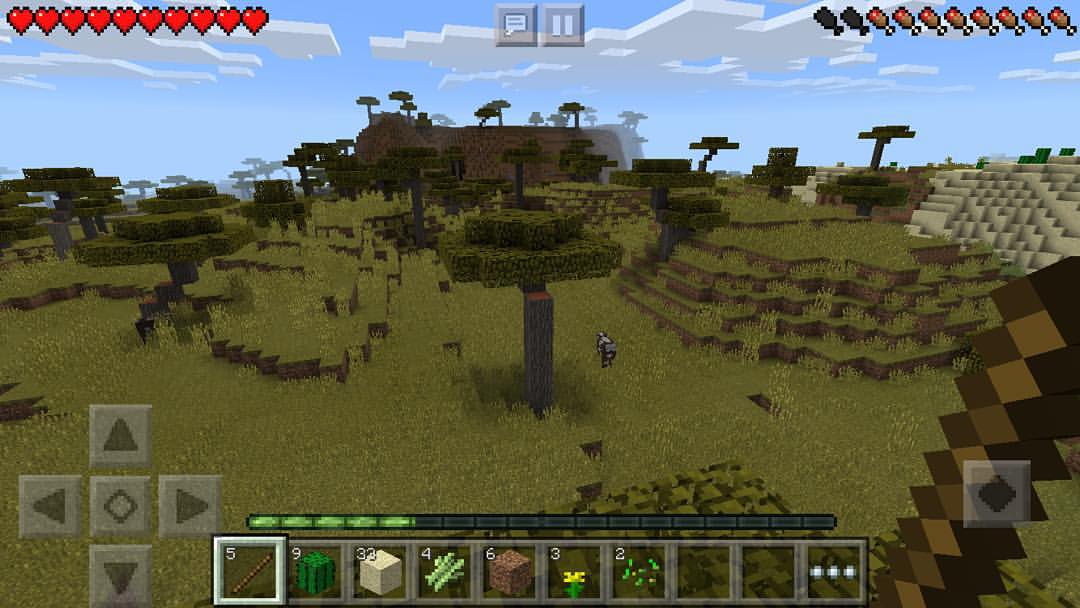This detailed screenshot from the game Minecraft showcases its iconic pixelated style. The in-game scene features a grassy plain with scattered trees, a cow grazing, and a cloudy sky overhead. The image is taken from a first-person perspective, with the player holding a brown wooden sword on the right side of the screen. The toolbar, found at the bottom of the screen, includes various items such as a stick, cactus, sand, and grass, each displayed with numbers indicating their quantity.

The heads-up display (HUD) includes key elements of survival in Minecraft. On the top left, the health bar is indicated by red pixely hearts, depicting the player's vitality. Adjacent to it, the hunger bar, comprised of food icons, displays the player's hunger levels. Additionally, the control arrows for movement are visible, indicating directions for up, down, left, and right.

Further, the interface includes a dialogue box and a pause button, as well as an enigmatic suggestion of wine glasses or similar icons on the right side of the screen, adding a mysterious touch to the game's environment.